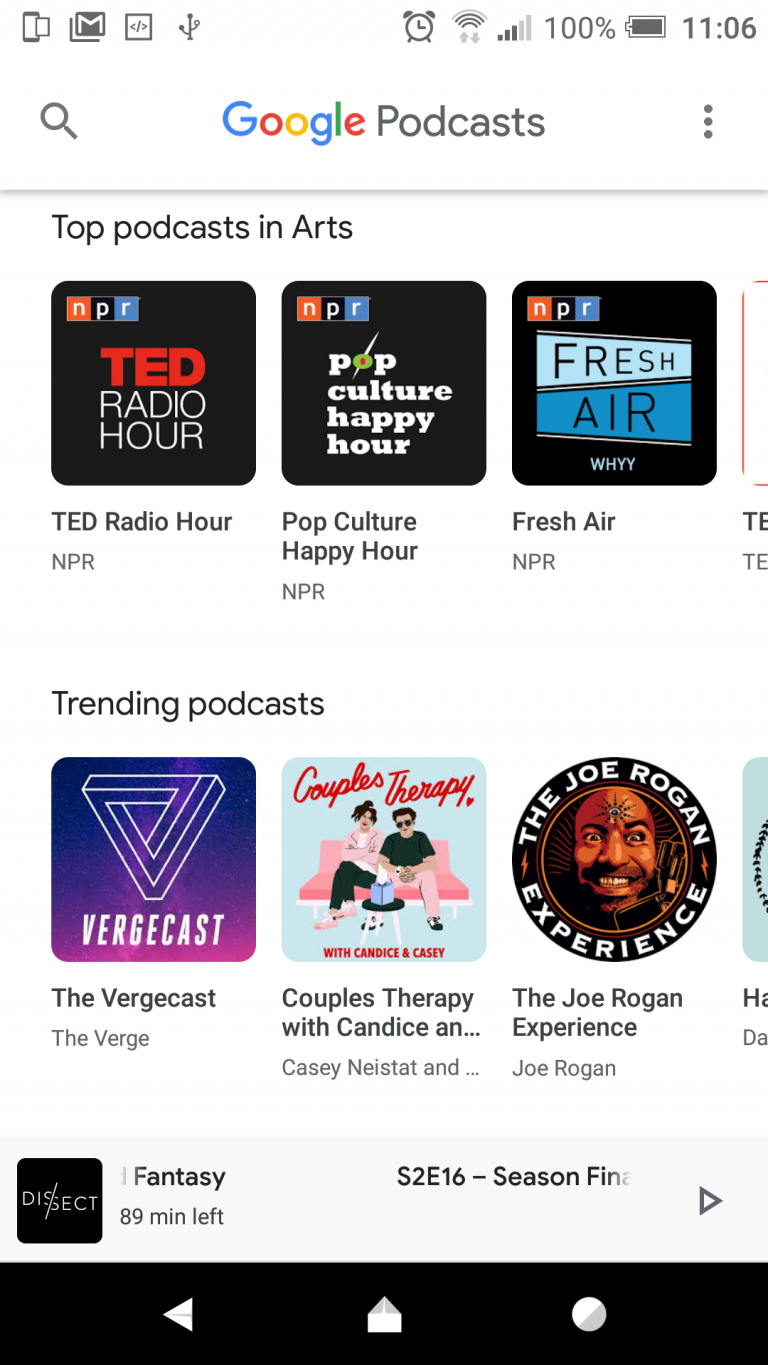This is a detailed screenshot of the Google Podcasts app from a smartphone. At the top right corner of the screen, there's a phone signal indicator, an 'M' emblem, another icon, a share symbol, and an earphone icon. Next to them, there's a clock showing the time at 11:06, followed by a speaker symbol, a five-bar signal indicator, and a battery status indicating 100%.

Directly below these icons, on the left side, a search icon can be seen. Centered on the screen, the Google logo appears in its iconic colors, followed by the word "Podcasts." Over to the right, there are three vertical dots next to a thin gray line.

Moving down the screen, the title "Top Podcasts in Arts" appears in black text. Listed beneath this title are three podcast recommendations, all from NPR: "TED Radio Hour," "Pop Culture Happy Hour," and "Fresh Air."

Further down, the title "Trending Podcasts" is displayed, highlighted in purple. Below this, three trending podcast recommendations are listed: "The Vergecast" with a purple icon, "Couples Therapy with Candice and Casey," featuring Casey Neistat and displaying a light blue background with a pink couch and a couple sitting on it, and "The Joe Rogan Experience," marked by its iconic round emblem with white letters around a dark circle.

At the bottom of the screen, a podcast episode named "Direct Fantasy, 89 Minutes Left, S2E16 Season Finale" is shown. A black line beneath the description includes icons for a left-facing arrow, an envelope, and a circle.